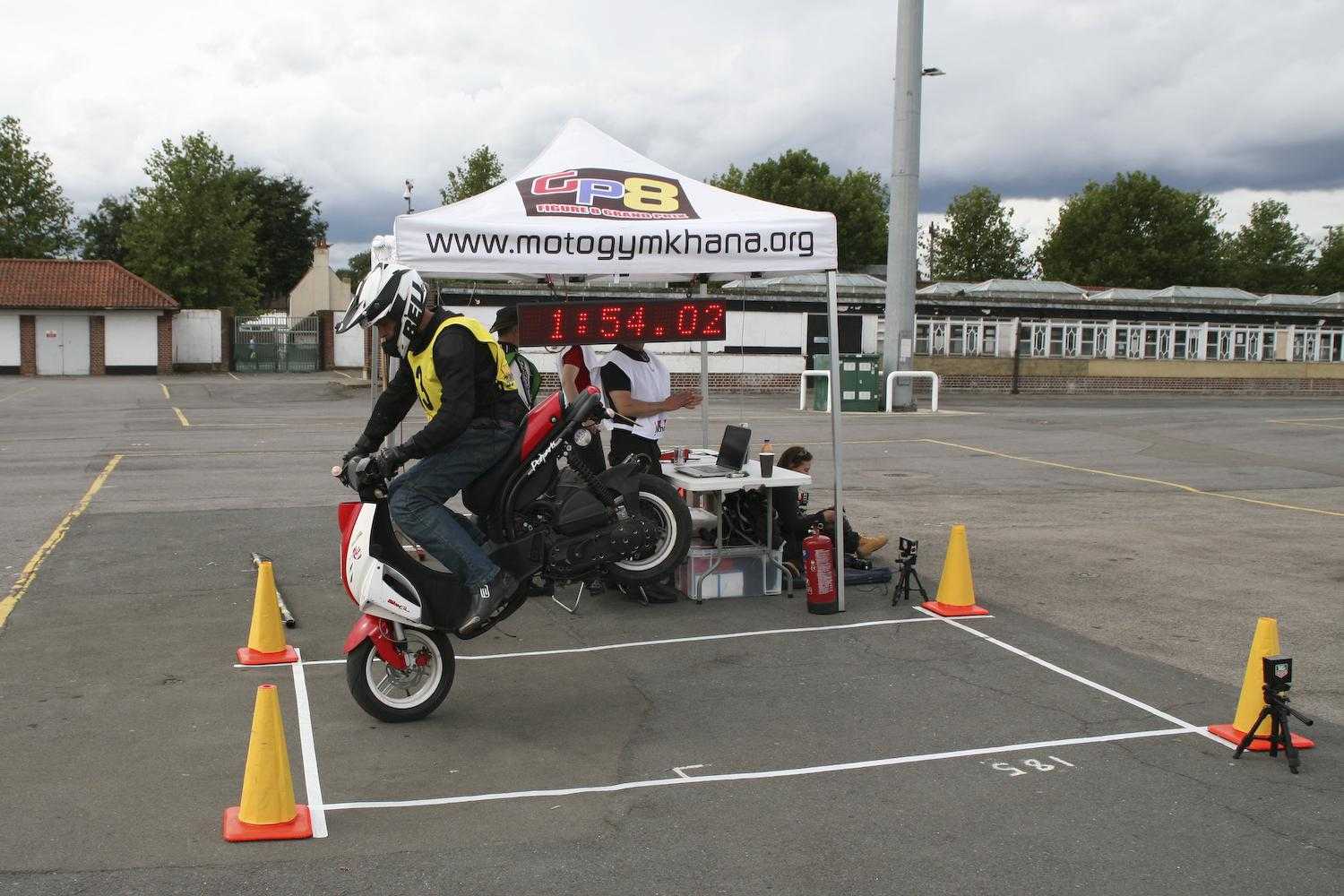The image captures an outdoor scene in a parking lot on a cloudy summer day, featuring a man skillfully balancing a red, white, and black motorcycle on its front wheel, with the back wheel lifted off the ground. The rider, dressed in a black top, blue jeans, black boots, and a yellow safety vest with a number, is also wearing a full white helmet. The practice area is delineated by white rectangular markings and orange and yellow cones.

In the background, there’s a canopy tent indicating the event is organized by "motojimkhana.org," a nonprofit. The tent shelters a table cluttered with equipment, a laptop, cameras on tripods, and a fire extinguisher. Two people in white vests stand under the tent, alongside a seated individual, all presumably keeping score. A digital timer beneath the canopy reads "1:54.02." The surrounding area includes deciduous trees, buildings, and garages, with a large light pole and an electrical box visible in the right background. The scene suggests an organized motorcycle skill competition, enhanced by the presence of a digital timer and marked practice area.